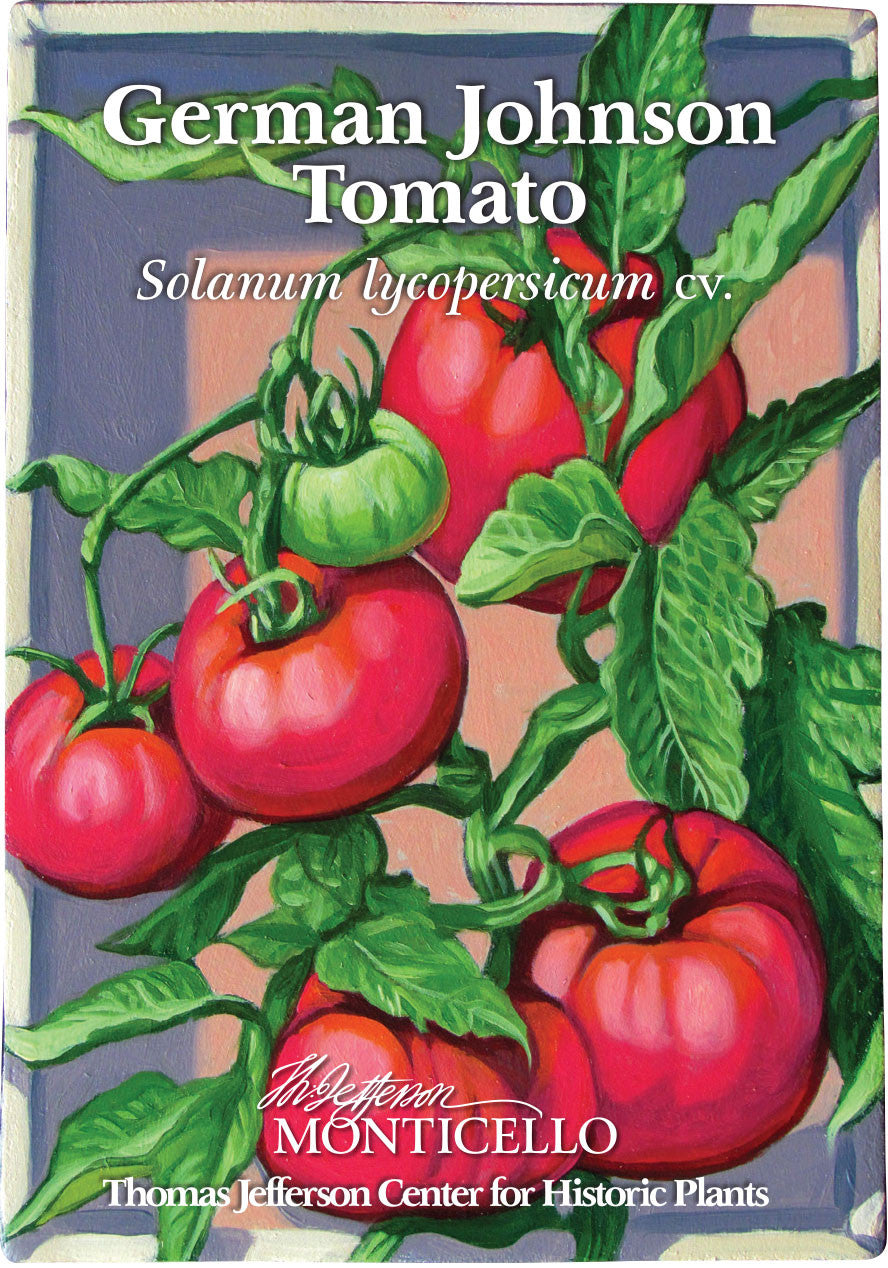The image depicts a detailed graphical illustration of a tomato plant, showcased on what appears to be either a seed packet cover or a poster, rendered in a watercolor art style. Against a purple and peach-colored background, five ripe red tomatoes and a single smaller green tomato hang from vibrant green vines with lush leaves, which seem to be part of a white trellis. At the very top, the text "German Johnson Tomato" is prominently displayed in white lettering. Below, the Latin botanical name "Solanum Lycopersicum C.V." is inscribed. Towards the bottom, there is a logo for "The Jefferson Monticello," followed by the text "Thomas Jefferson Center for Historic Plants." The top border of the image is light green, adding a subtle, harmonious contrast to the overall design.